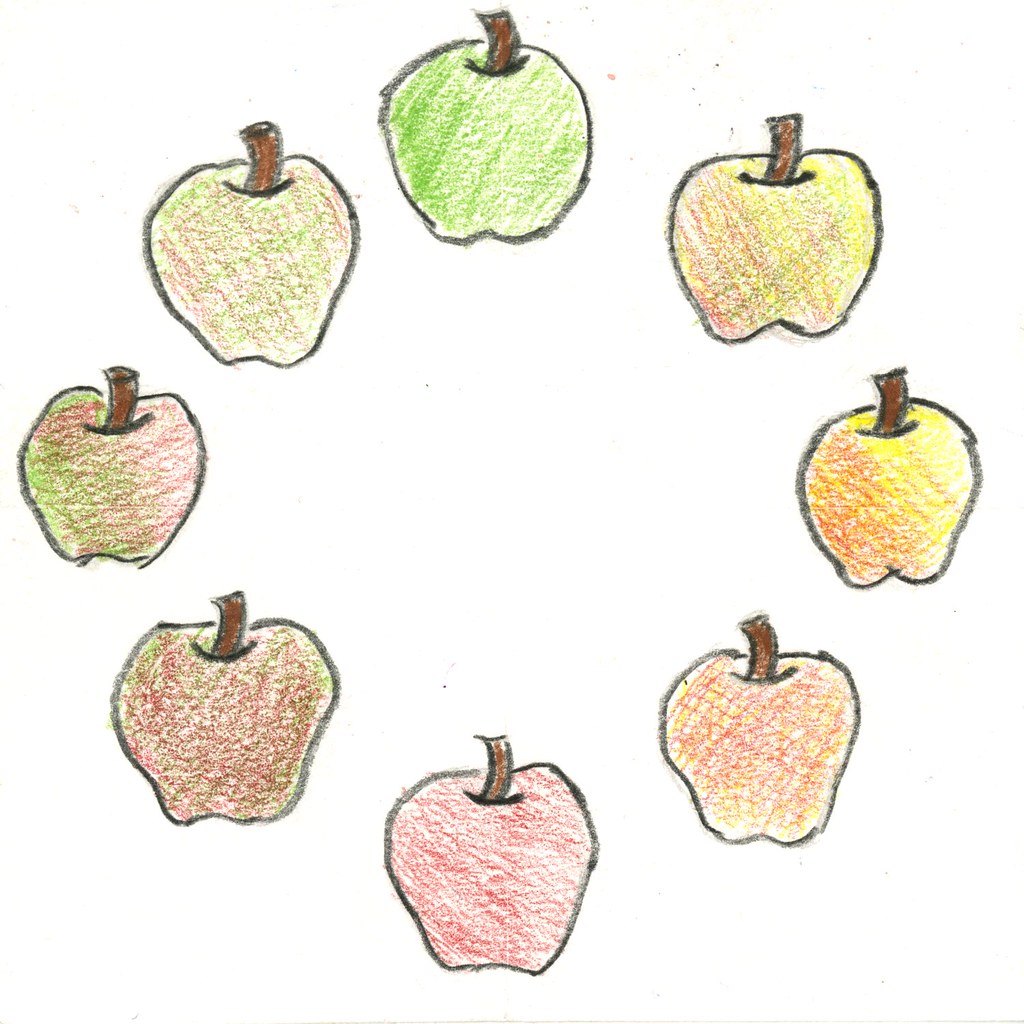This is a detailed colored pencil drawing on white paper, featuring eight apples arranged in a perfectly symmetrical circle with no background. Each apple is meticulously illustrated, showing a variety of colors—green, red, and yellow—with subtle blending. At the top, a green, round apple with a brown, slightly curved stem sets the starting point. Moving clockwise, the next apple features a mix of green and red, followed by another apple that is primarily red with hints of green. Further down, around the 5 o’clock position, there is a predominantly red apple, transitioning to an even lighter red apple with pinkish tones at the bottom of the circle. Continuing up, a pinkish apple with some yellow highlights appears, leading to a mostly yellow apple with red accents on the right side of the circle. The final apple, located at about the 1 o’clock position, has a yellow base with touches of red and green. All apples are strikingly similar in shape and size, unified by their short, stubby brown stems. The meticulous use of colored pencils creates a soft texture, enhancing the organic feel and vibrancy of each apple within the composition.